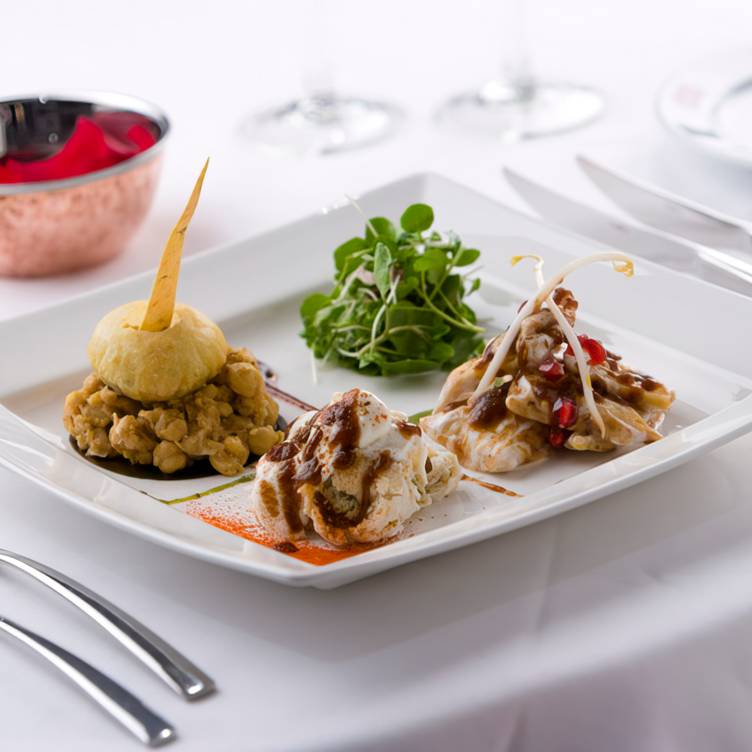A photograph captures an elegantly set table with a white tablecloth, showcasing a rectangular white porcelain plate at the center foreground. The plate is artfully arranged with various dishes, including a clump of creamy white mashed potatoes adorned with lines of brown gravy situated at one corner. Directly diagonal to the mashed potatoes is a small heap of fresh green salad leaves. Adjacent to the mashed potatoes is a fancy, dark brown clumped dish, possibly a medley of different foods. Nearby, there is a bun-like dish with pieces of chicken and green bean sprouts on top. The right side of the plate also features a visually appealing assortment of meat dishes. In the foreground to the left, the ends of two pieces of silverware, likely knives, are visible. Behind the plate, slightly out of focus, stands a stainless steel and copper-toned bowl lined with a vibrant red cloth. The backdrop is completed with an array of wine glasses, contributing to the sophisticated tablescape.